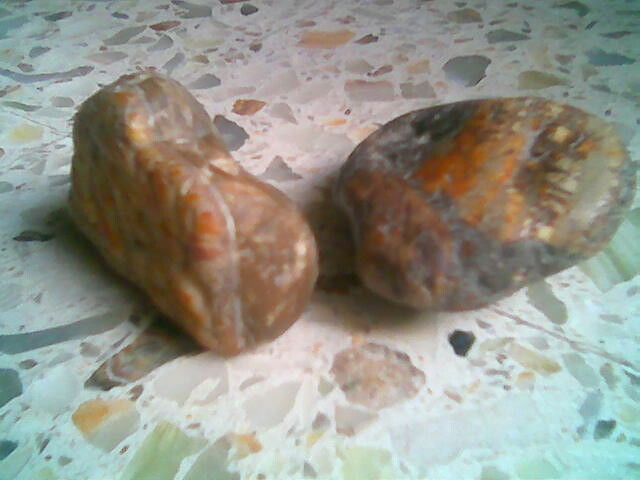This image features two prominently displayed, bumpy rocks set on a textured surface inlaid with various small stones of different hues, including blues, reds, greens, and clears. The surface itself is flat, possibly resembling a concrete slab or table. The rock on the right is notably oval or egg-shaped, exhibiting a mix of earthy tones such as dark blacks, browns, and reds, with some polished, reflective areas. Its distinctive feature is a white or silverish seam running around its lower part. The rock on the left, oriented in an upright position, is described as parfait-shaped or oblong with a noticeable dent in the middle. It showcases a blend of colors including light brown, orange, and some gray. The overall scene is a bit out of focus around the edges, adding a dreamy, slightly dark ambiance to the setting.